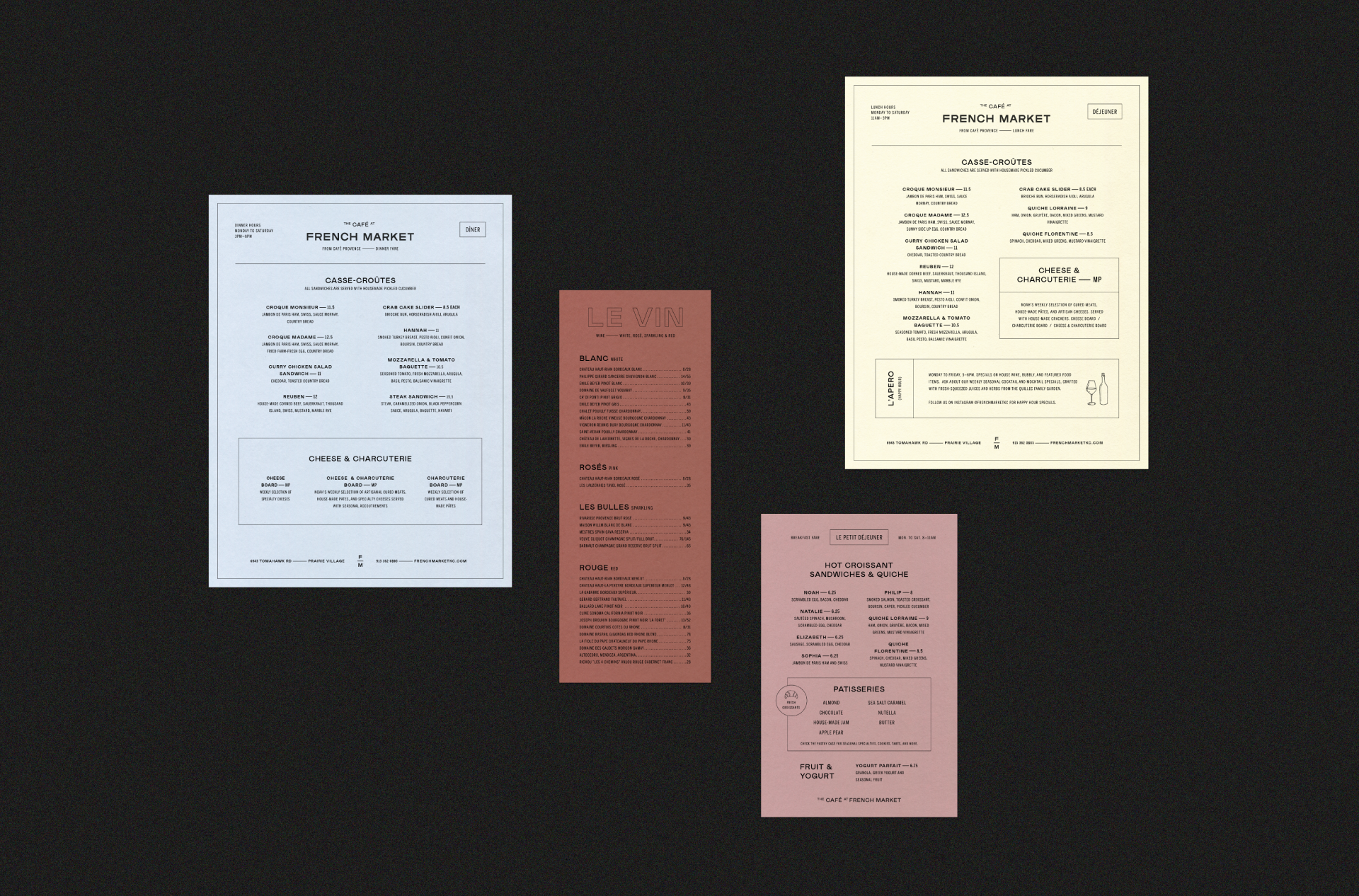Against a dark background, this image showcases four pieces of paper with distinct colors and text. The first piece on the left is a white rectangle labeled "French Market" at the top, followed by a title "Cassez-Crutes." It features black text in two columns, with most of it being too small to read except for a section indicating "cheese" and another foreign word. Beneath that are three sections of additional black text. 

Next to it, a dark orange paper prominently displays "LEVIN" in outlined letters at the top. Below, it lists items alongside their prices, divided into four sections. 

In the upper right corner, a yellow piece of paper, also titled "French Market" at the top with a bar underneath, mirrors the layout of the first paper. It includes "Cassez-Crutes" followed by two columns of text, and a notable section indicating "cheese." Below this information is a rectangle spanning the width of the page with further black text.

The final paper, featuring a purple background, is labeled "Hot Croissant, Sandwiches, and Quiche," and includes two columns of text too small to read, with a below section titled "Pastries" listing two columns of pastries. Additionally, on the bottom left side, it mentions "Fruit and Yogurt."

This detailed arrangement of papers collectively presents menus or lists, each with distinctive color backgrounds and titles, with "French Market" appearing twice, emphasizing its relevance.